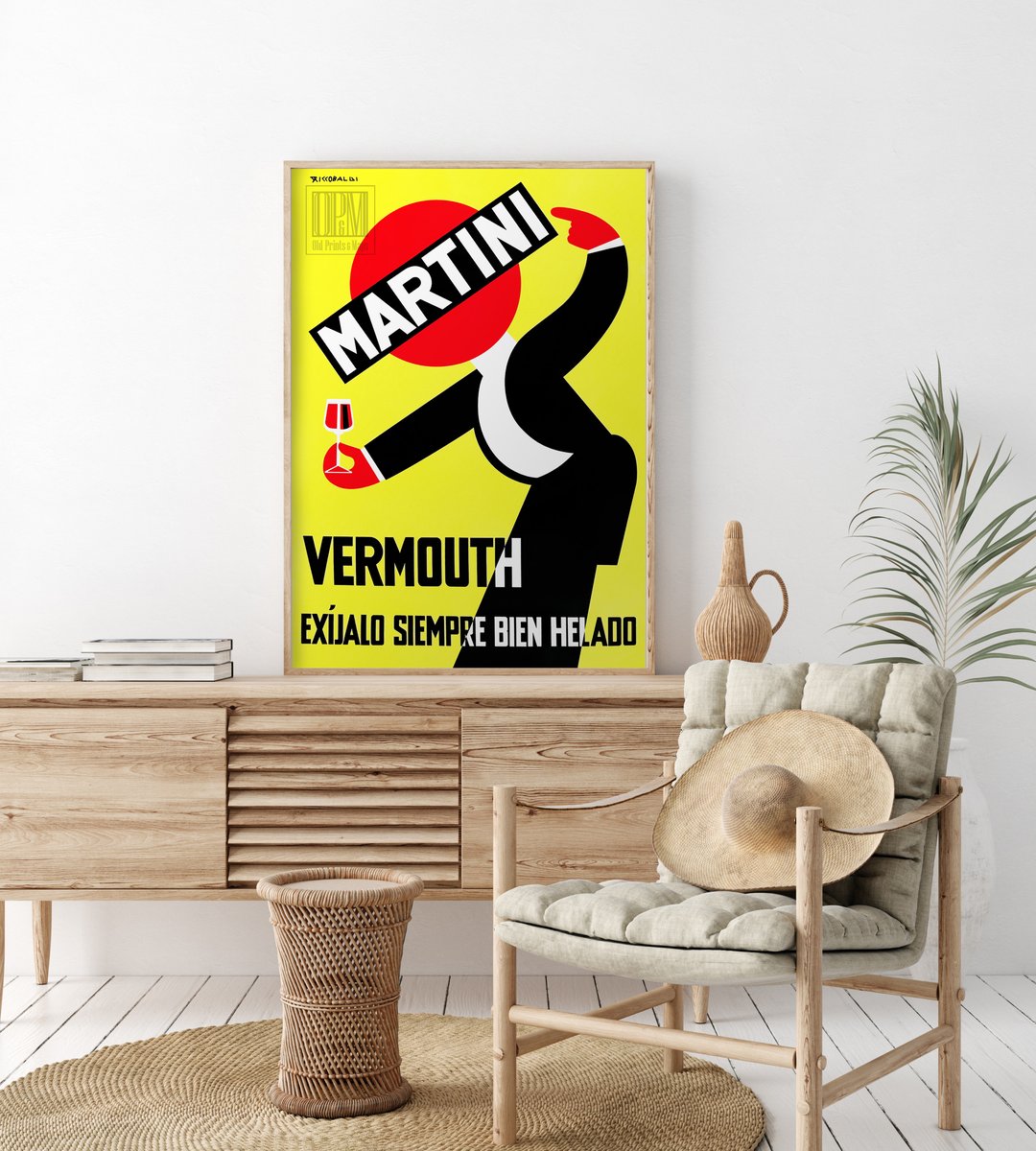This photograph captures a stylish living room corner dominated by a large, eye-catching poster from the brand Martini. The poster, primarily yellow with vibrant flashes of red, black, and white, features a Spanish phrase that reads "Existo Siempre Bien Gelado" at the bottom. It portrays a man with a large, red circular face pointing towards the brand name that is displayed prominently across his face. The man is also holding a glass filled with a red drink, presumably vermouth, in his left hand, while crouching.

The setting is a rectangular wooden table, adorned with a few books and a brown vase, exhibiting a blend of boho chic and pastel colors that make the vivid poster pop. The table sits against a wall painted white, resting on a light brown, circular woven rug. To the left of the table, a wooden chair with a tapered design holds a large flat brown hat and a gray cushion, complementing the natural wooden and white tones of the room. Nearby, a cylindrical woven basket with frilled edges contains dried green fronds, adding a touch of rustic charm. Additional accents include a cylindrical drum-shaped table and a variety of wooden furniture, creating a warm, inviting, and well-decorated living space.